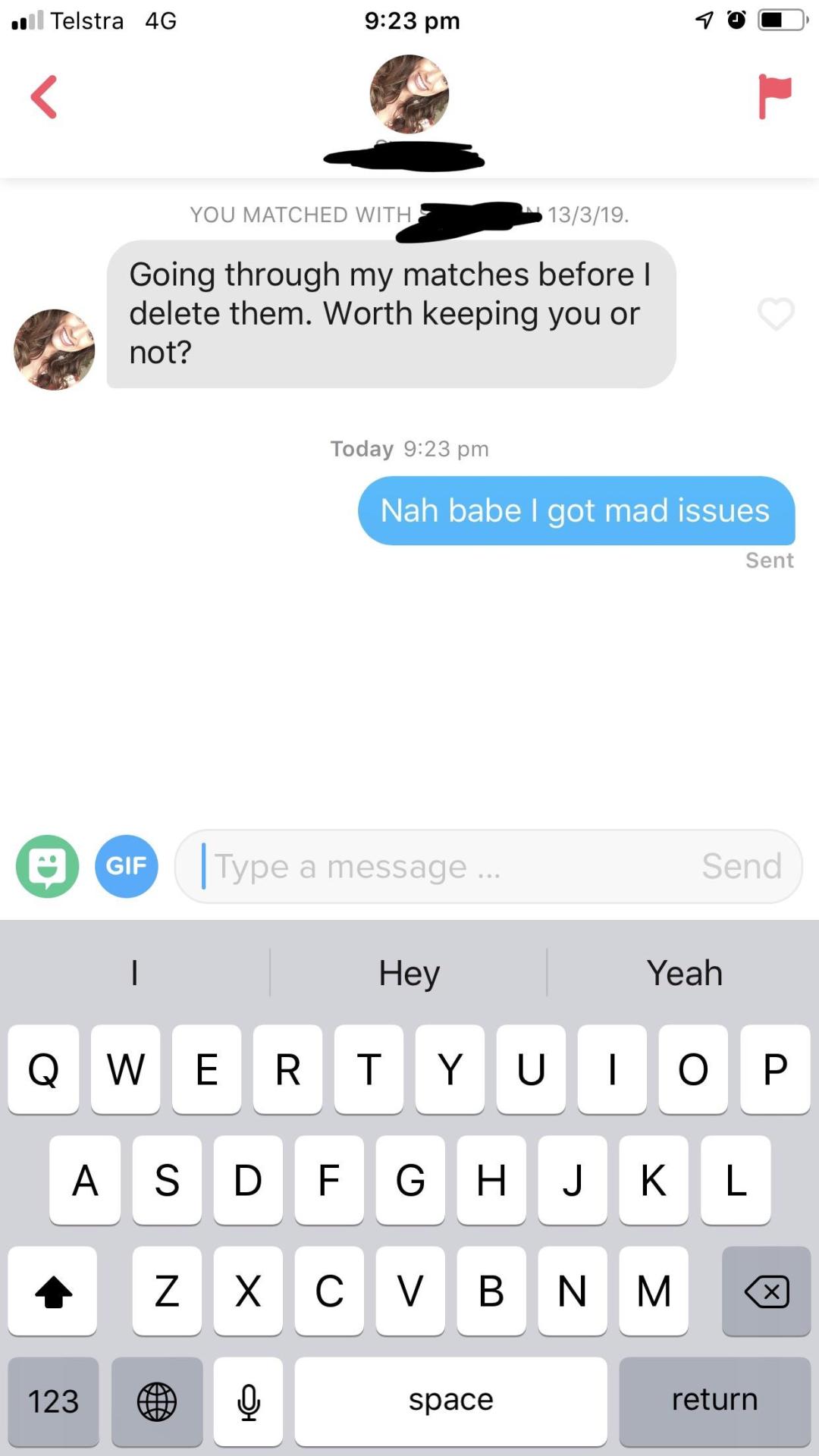This screenshot captures a text message conversation on a mobile dating app interface. At the top, the status bar displays the Telstra carrier name, 4G connectivity, the time (9:23 PM), and various icons indicating location usage, an alarm set, and a battery at approximately fifty percent charge.

In the app section of the screenshot, a profile picture of a smiling girl with curly hair is centered between a back button on the left and a red flag icon on the right. Just below this, text reads, "You matched with [Name] 13/3/19." This is followed by her message in a gray speech bubble, stating, "Going through my matches before I delete them. Worth keeping you or not?"

The reply, timestamped today at 9:23 PM, appears in a blue speech bubble: "Nah babe, I got mad issues." The keyboard is visible at the bottom, and directly above it sits the message input box where new messages can be typed. To the left of the message input box, there is a blue gift button and a blue picture button, indicating options to send gifts or photos. The standard phone keyboard is ready for further typing.